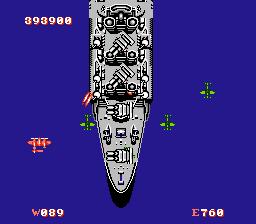This image depicts a dark blue square featuring various numbers and letters in three of its corners. In the upper left corner, the number "393900" is displayed prominently in white with a subtle red outline. In the lower left corner, a red "W" accompanied by the numbers "089" in white can be seen. The lower right corner features a red "E" followed by the number "760" in white.

Within the blue area of the square, there is a detailed illustration of a battleship surrounded by four airplanes. Among these aircraft, three are green, each equipped with a single propeller. In contrast, there is one red airplane that stands out due to its dual propellers, each positioned on either side of the central fuselage.